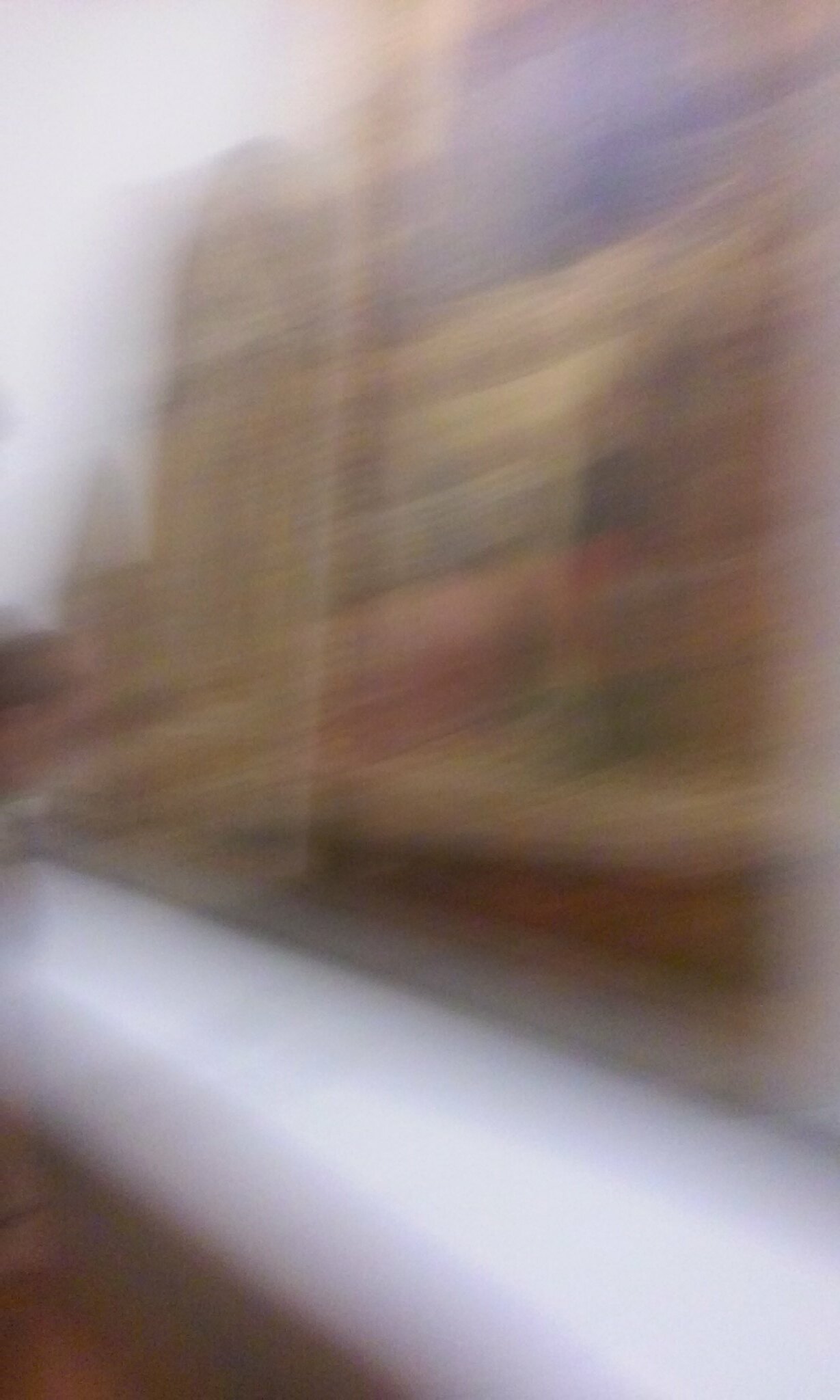This image is notably blurred, suggesting it might have been taken from a moving vehicle, possibly a train or a car. In the foreground, there is a vague white, possibly cylindrical section that might be part of a window ledge or sill, indicating the photo could be capturing a reflection. The upper portions of the image feature a washed-out white area, likely representing a cloudy or overcast sky. Towards the left, there's a distinct yet faded square structure with an upward triangular roof, giving the impression of a building. Adjacent to this, another building with a rounded, brownish hue is visible. Further right, a structure exhibits hints of red in its front and more brown tones in the background. Despite the overall blurriness, the repetition of triangular roofs and the combination of brown and red hues in the buildings suggest an urban landscape swiftly passing by in a motion-blurred capture.